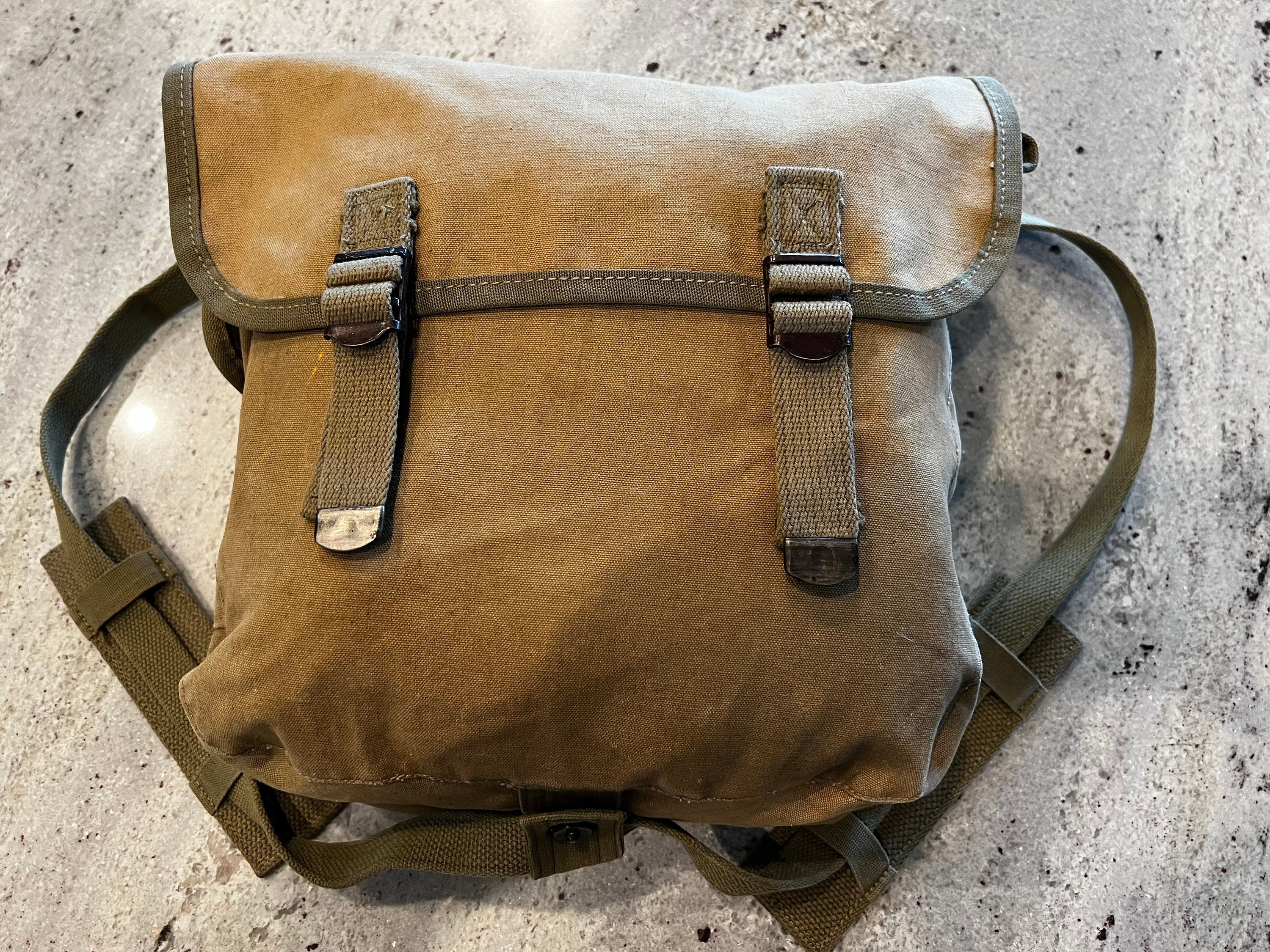The image displays a close-up of a brown square-shaped bag, lying on a blended light brown and light gray stone ground, with more brown hues on the left and lighter gray on the right, accented by tiny black marks scattered throughout. The center of the image is dominated by the bag, which is medium brown with dark brown, mocha-colored stitched trim. It features two vertical buckles descending from its flap, one on each side, and a greenish-brown strap with padded sections for comfort. The flap can be lifted, suggesting the bag is filled, giving it a slightly bulky appearance. The ground appears cemented with small gaps and specks of brown and black, enhancing the rugged, utilitarian aesthetic of the scene.